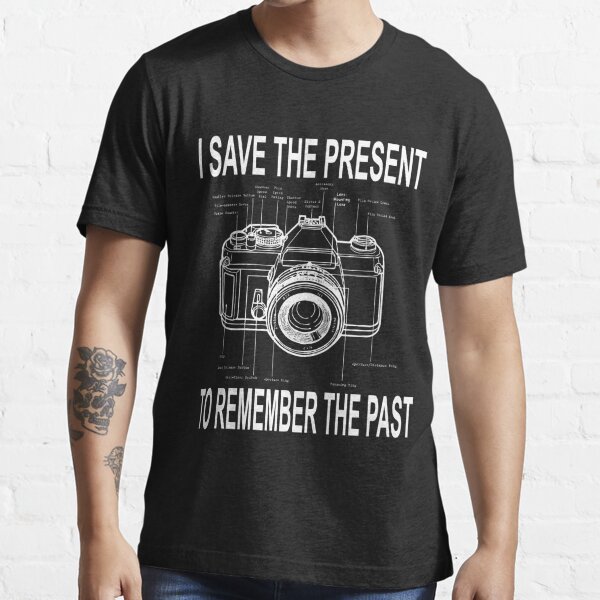The image is a color photograph in portrait orientation, featuring a Caucasian man, likely in his 20s, modeling a dark grey, almost black, crewneck t-shirt with short sleeves. The photo captures him from the bottom of his chin to about mid-hip, showing the very top part of his blue jeans. Prominently displayed on the t-shirt is a bold white text reading, "I save the present," above an illustration of a camera depicted in grey and white, shown from the front, focusing on the lens. Below the camera, another bold white text reads, "to remember the past." The camera graphic includes multiple small labels pointing to different aspects of the camera, though the text on these labels is not legible. The man has a distinctive black skull tattoo with a rose emerging from the top on his right forearm, with the design extending from his antecubital space to near his wrist. His left arm is also visible. The background of the image is a white-painted brick wall, providing a minimalist yet textured backdrop, enhancing the focus on the subject and the t-shirt. This image exemplifies photographic representationalism and realism, characteristic of product photography aimed at highlighting the details and message of the t-shirt design.